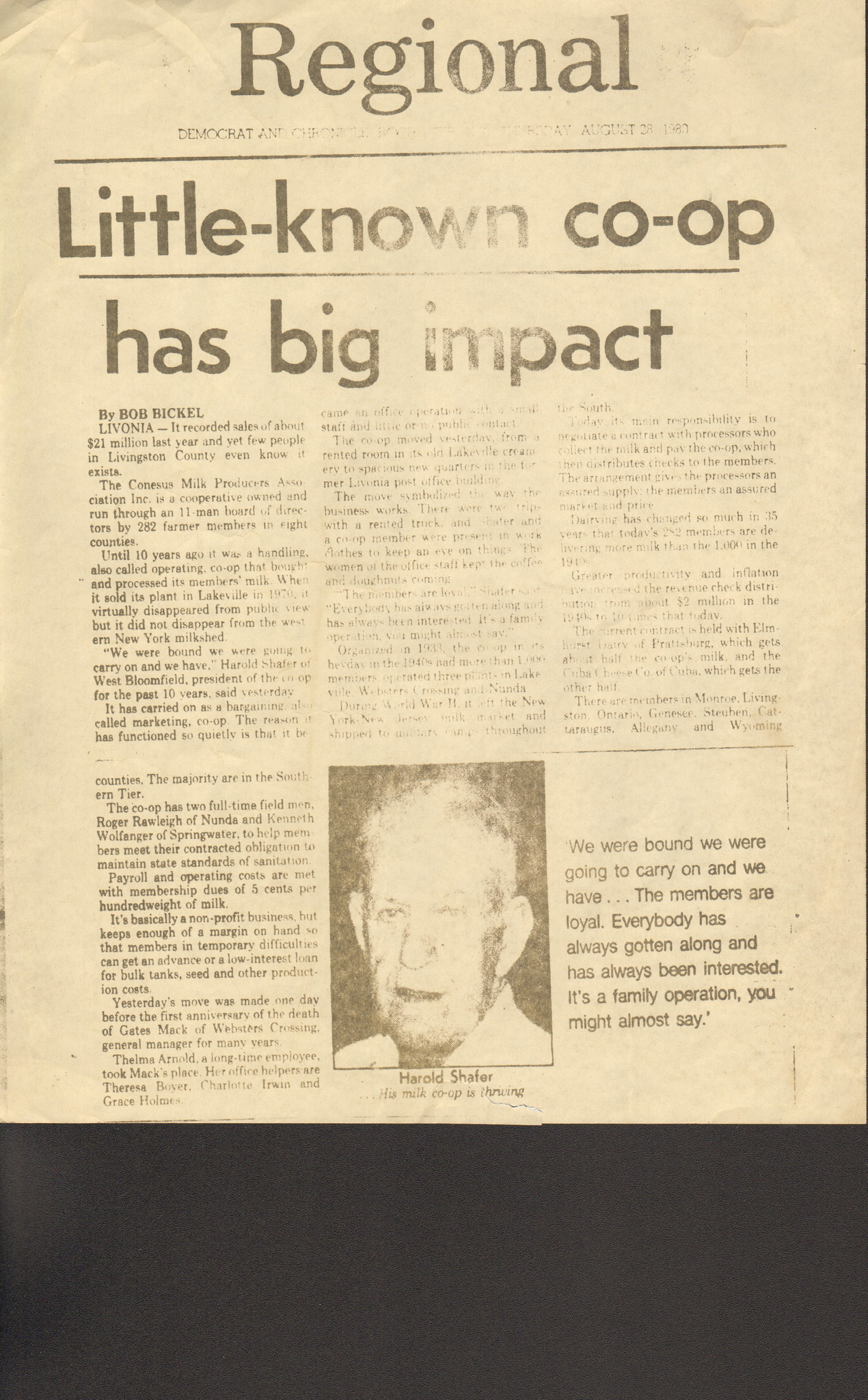The image displays a very old newspaper or magazine page with an aged yellow background. At the very top center, large black text reads "REGIONAL," and beneath it, some smaller text, including partially readable words like "DEMOCRAT" and "AUGUST." The headline of the article is "Little Known Co-op Has Big Impact," authored by Bob Rickle from Livonia. The story highlights the co-op's recorded sales of about $21 million last year, despite its low profile in Livingston County. The article is composed of three paragraphs, which are difficult to read due to fading. Below the text is a black-and-white photograph of an elderly man looking towards the camera, identified as Harold Schaefer with a caption mentioning the thriving milk co-op. On the right side of the photograph is a caption under the third column quoting, "we were bound, we were going to carry on, and we have... the members aren't loyal, everybody has always gone along, and has always been interested, it's a family operation, you might almost say."